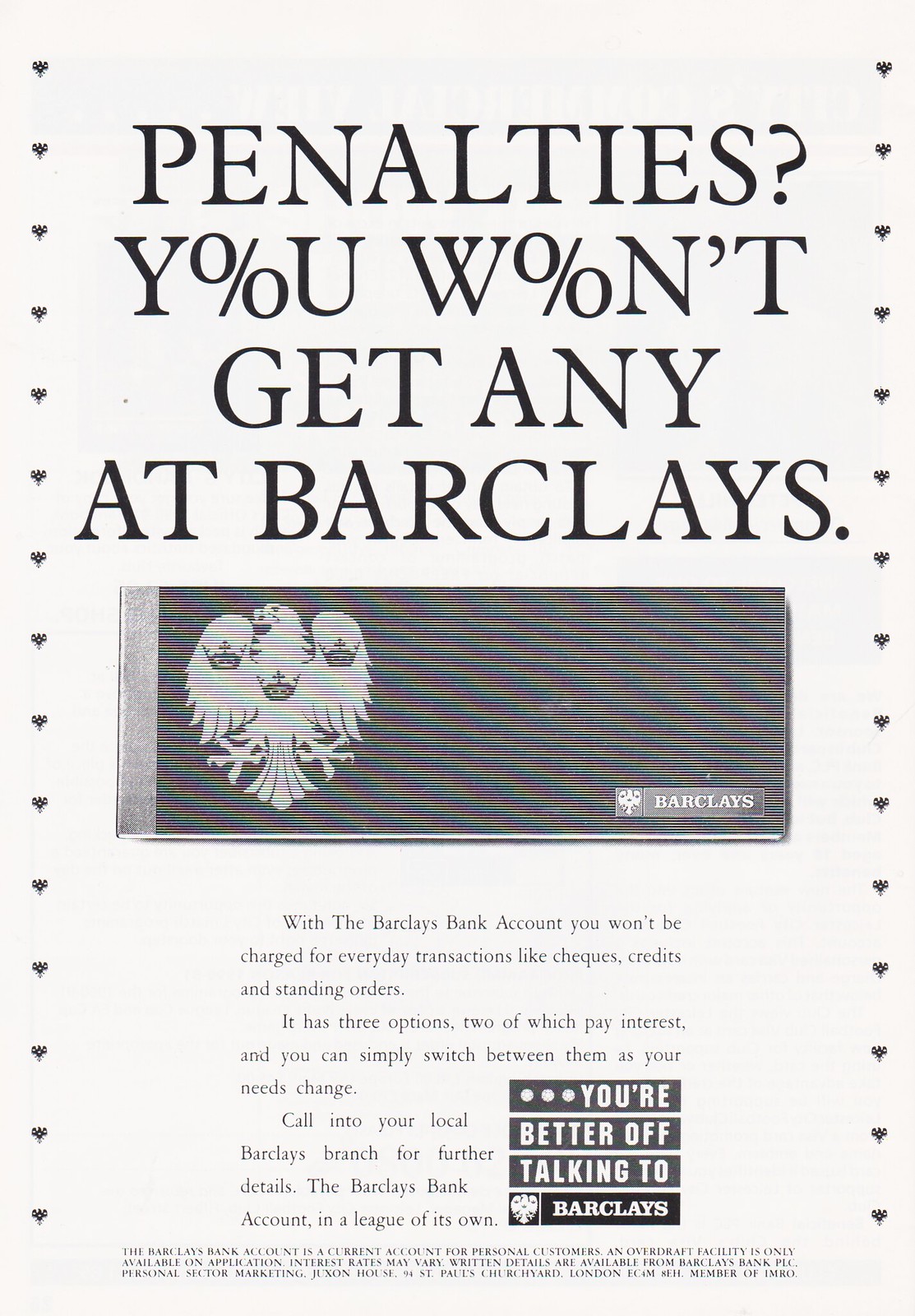This vintage-style print ad from Barclays, suitable for a magazine, combines clean graphics and precise typography against a beige background. Dominated by black-and-white elements, it features a prominent headline in all caps: "PENALTIES? YOU WON'T GET ANY AT BARCLAYS," where the O in "YOU" and "WON'T" is cleverly replaced with a percentage sign. 

The ad is bordered by vertical rows of tiny white Barclays eagle emblems with three crowns on their bodies, lending an air of sophistication. Central to the design is a horizontal depiction of a checkbook cover, dark gray in color, displaying the Barclays eagle logo in white on the left and the Barclays logo in gray with white lettering on the bottom right corner.

Below, a detailed paragraph elaborates on the advantages of the Barclays bank account, highlighting that everyday transactions such as checks, credits, and standing orders incur no charges. It offers three interest-bearing options, easily switchable based on changing needs. The call-to-action invites readers to visit their local Barclays branch for more details.

The lower section reiterates the value proposition: "YOU'RE BETTER OFF TALKING TO BARCLAYS," set against a black backdrop with white text. The ad concludes with fine print about account terms, including overdraft facilities and a disclaimer on varying interest rates. Contact information is provided for further inquiries, underscoring Barclays' commitment to customer service.